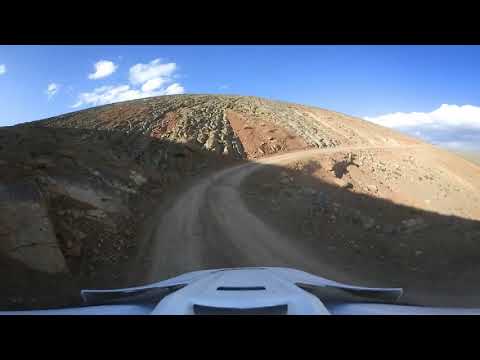The image depicts a dirt path winding along the side of a bare mountain hill, carving its way from the bottom center to the right edge of the frame. The scene is framed by thick black borders at the top and bottom, creating the impression of a view from within a vehicle, possibly a motorcycle or another vehicle, given the silver hood ornament visible at the bottom center of the image. The path initially splits into two before merging and curving to the right. The left side of the hill shows sparse patches of green amidst the predominantly brown, barren surface, while the right side appears mostly dirt with hints of green. Shadows cast by the sun stretch across the foreground from the left to the bottom right, contrasting with the sunlit terrain in the background. Above the hill, the sky is a delicate blend of blue and white clouds, adding a serene backdrop to this rugged landscape.